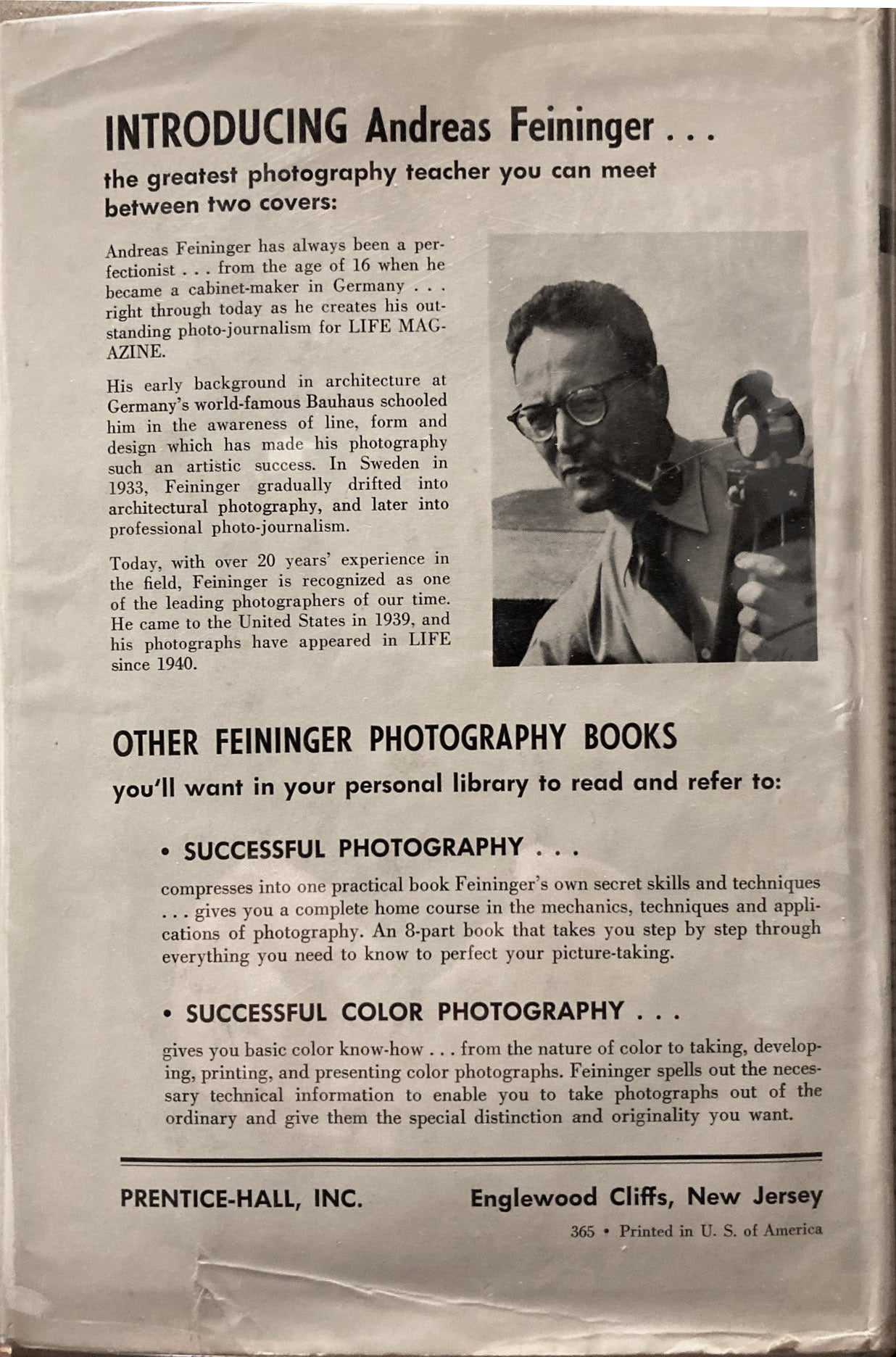This black and white photograph of a torn page from an older textbook appears to be an advertisement introducing Andreas Feininger, hailed as "the greatest photography teacher you can meet between two covers." The ad features a portrait of Feininger wearing glasses and a shirt and tie, smoking a pipe while holding a camera. The page describes Feininger's illustrious career, from his early days as a cabinet maker in Germany to his architectural education at the Bauhaus, and his evolution into a renowned photojournalist for Life Magazine since 1940. The text emphasizes his thorough understanding of line, form, and design, which contributes to his photographic artistry. Additionally, the page promotes Feininger's photography books—"Successful Photography" and "Successful Color Photography"—highlighting their practical, step-by-step guides to mastering both black and white and color photography. As indicated at the bottom, this page was published by Prentice Hall, Inc., based in Englewood Cliffs, New Jersey, and is marked with the page number 365. The paper shows signs of age, with grayed tones and slight tears at the edges.